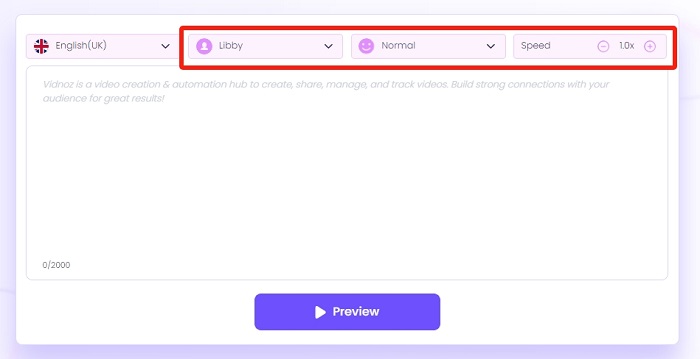This horizontal screenshot features a user interface captured from a computer screen. The image showcases a purplish and whitish ombre border that darkens at the bottom and lightens at the top, with a similar gradient effect on the sides. 

In the top left corner, a circular icon displays the UK flag next to the text "English (UK)." Below this, there are interactive elements with arrows that allow selection of various options. A prominent red rectangular box highlights three clickable options: "Libby" with a graphic image of a person's face, a smiley face icon labeled "normal," and the text "speed 1.0x."

Centrally, a white box with a gray border provides information about "VidNoz," describing it as a video and automation hub designed to create, share, manage, and track videos, helping to build a strong connection with the audience for better results. The text within this box indicates a character limit, displaying "0 / 2000."

At the bottom of the image, a blue button with a white right triangle and the word "Preview" invites the user to preview their content.